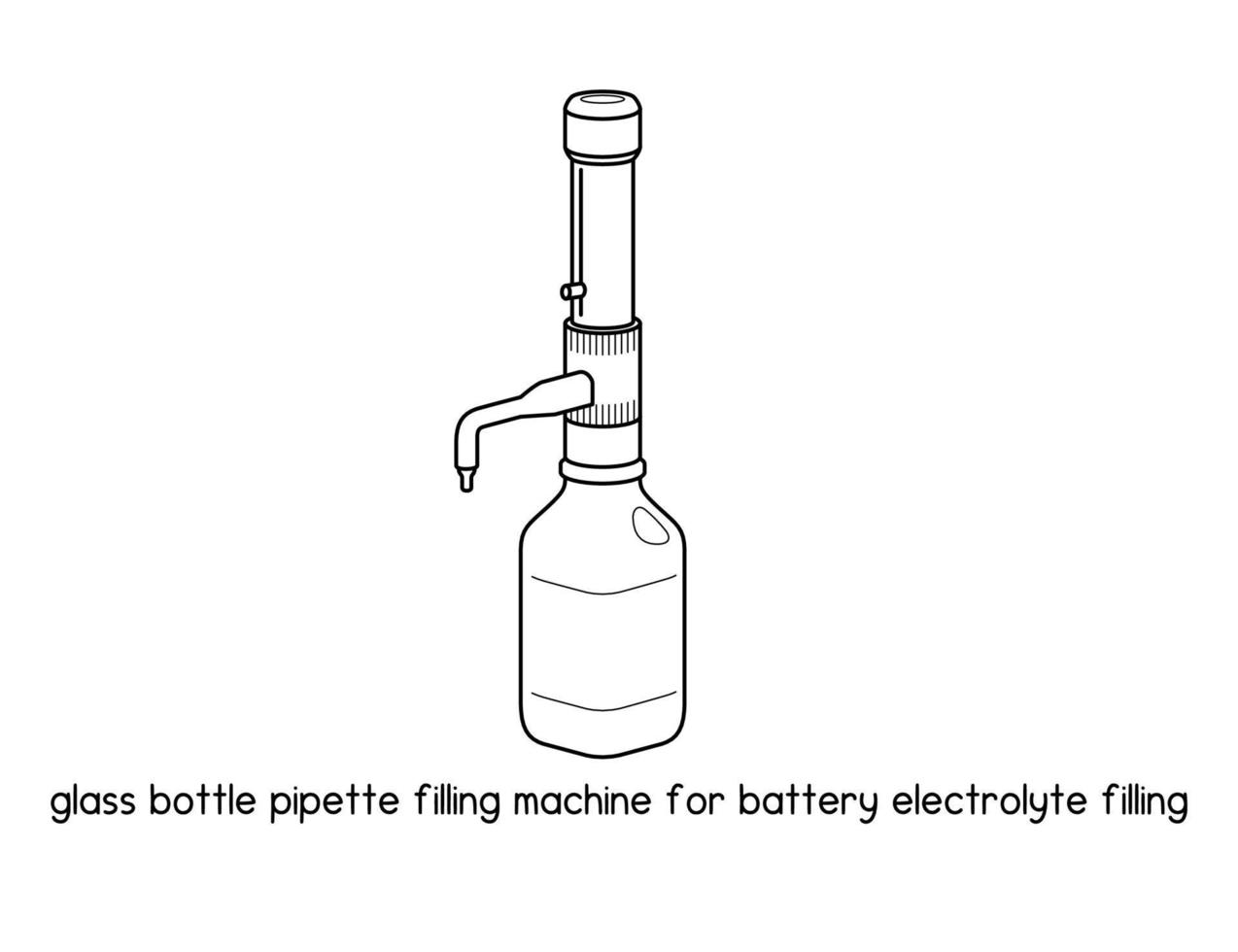The image illustrates a black-and-white sketch of a glass bottle pipette filling machine designed for battery electrolyte filling. The text, in small black lowercase font at the bottom, reads: "glass bottle pipette filling machine for battery electrolyte filling."

The central focus is a white glass bottle with a rounded square shape. At the bottle’s opening, there is a horizontally extending cylindrical spigot attached, designed to dispense liquid. This spigot features a 90-degree bend directing downward for precise filling.

Above the spigot, a vertically mounted tube with a handle is visible, ending in a circular opening. Additionally, near the bottom of the bottle, there is a holding reservoir for the liquid. The simplistic, detail-oriented sketch is rendered entirely in black against a white background, emphasizing the mechanical design and functionality of the filling machine.